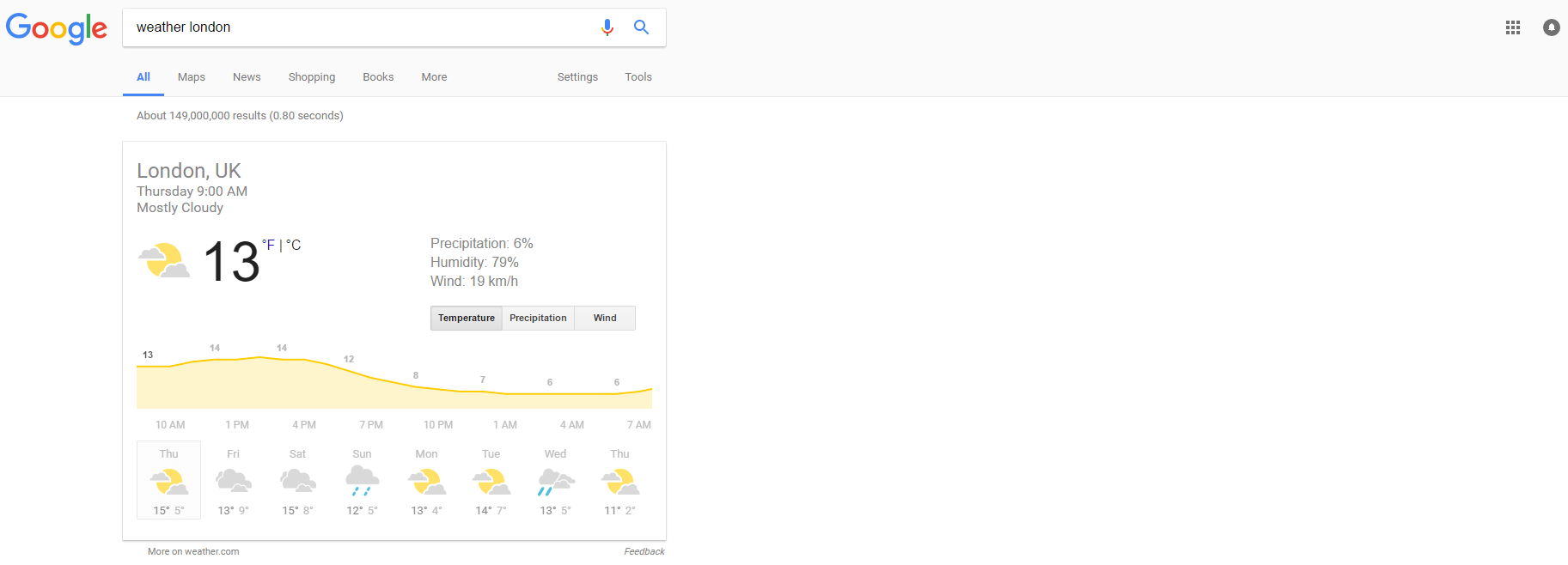A detailed weather report for London, UK appears in a Google search. The image prominently features a forecast for Thursday at 9 a.m., indicating that the weather is mostly cloudy. An icon of the sun peeking through clouds visually represents the forecast. The current temperature is displayed as 13 degrees Fahrenheit, with additional details showing 6% precipitation and 79% humidity. A line graph illustrates the temperature trend for the day, starting at 13 degrees at 10 a.m. and rising as the day progresses, before gradually declining overnight. A week-long forecast is also available, covering Thursday through the following Thursday, with daily temperature readings. The interface includes a microphone for voice input, a magnifying glass likely for search functionality, and a series of dots on the right side, which provide access to other Google applications such as Google Docs and Google Sheets.